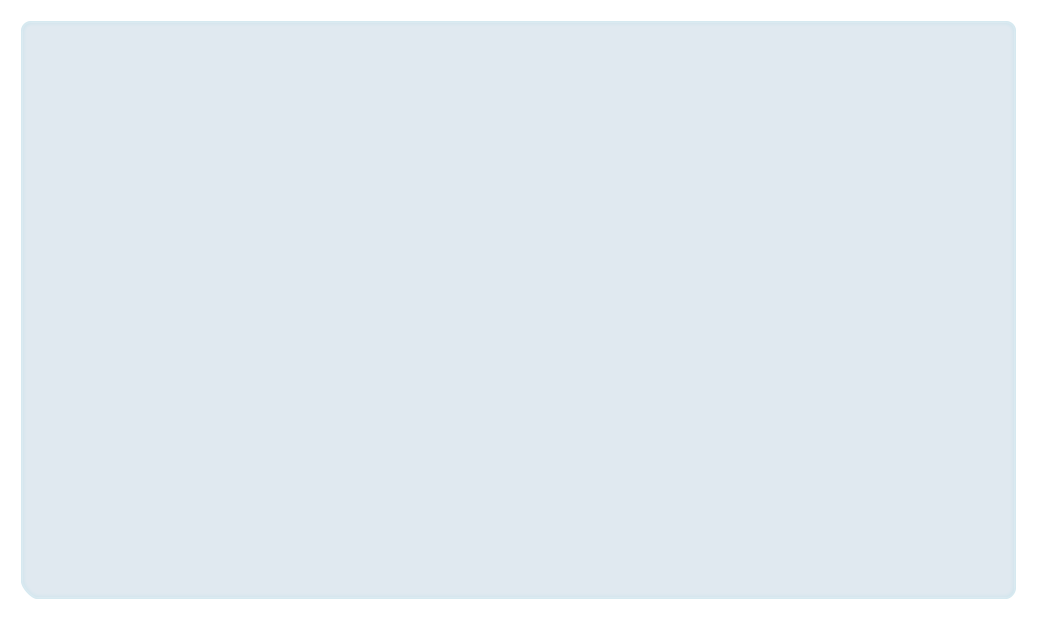The image displays a blank, light gray rectangular box, akin to the dimensions of a typical webpage viewed on a computer monitor. The box is devoid of any text or images, enclosed within a faint, slightly darker gray border. The simplicity of the scene suggests either an image that failed to load properly or an intentionally minimalist design. The overall visual is marked by the stark absence of content, providing a neutral, empty canvas.